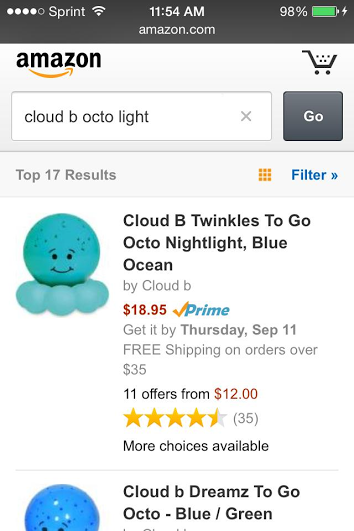Here is a cleaned-up and detailed caption for the image described:

---

The image depicts an Amazon store page as viewed on a smartphone. At the very top of the screen, there are four indicator dots, the first and third dots are filled indicating their status, while the second and fourth dots are open. To the right of these dots, the word "Sprint" is displayed in white text. Adjacent to "Sprint" on the right, there is a fully filled Wi-Fi signal icon. In the center of the top bar, the time reads "11:54 AM." Further to the right, the battery status indicates 98% with a nearly full, green battery icon displaying a charging symbol (lightning bolt).

Immediately below the status bar is the Amazon header. It starts with the Amazon logo on the left, featuring the word "Amazon" in black, with a smiley arrow from "A" to "Z." On the far right of the header, there is a shopping cart icon with five dots indicating items in the cart, arranged with three dots on the top row and two on the bottom row.

Further down is a search bar showing the text "cloud, B, Octo, light," with an "X" on the right side to clear the search field and a "Go" button to initiate the search. Below the search bar, a light gray background contains the text "Top 17 results" in gray on the left and an orange icon followed by a blue icon with a double arrow to the right.

The first product displayed below this line is a blue octopus night light. The product name reads "Cloud B Tranquil Octopus Night Light," and further details include the price of "$18.95," eligibility for Prime shipping with a promise of delivery by "Thursday, September 11th," and a note for "Free Prime Shipping" on qualifying orders.

---

This detailed caption provides a clear, structured description of the elements found in the image of the Amazon store page on a smartphone, including interface specifics and product details.